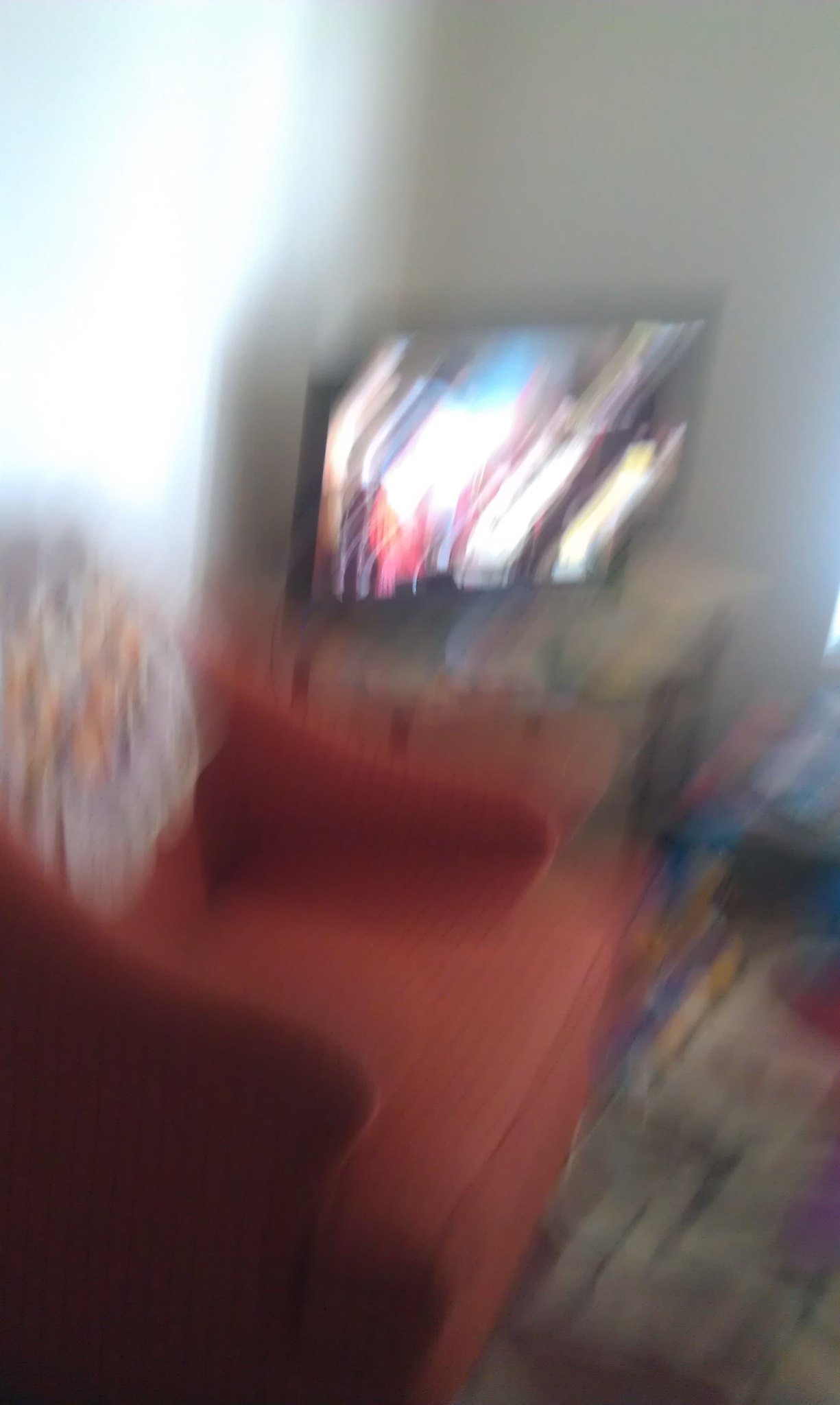In this blurry image of a living or TV room, we observe a space bathed in daylight, with sunlight streaming in against the white walls. Central to the scene is a red cloth sofa, covered with an embroidered cloth, displaying refined detail despite the overall blurriness. To the left of the sofa sits an orange or rust-colored reclining chair, potentially made of cotton, adorned with a multicolored pillow draped over the back. Dominating the center of the room's attention is a flat screen television, which is switched on but too blurred to reveal its content. The TV rests on a black TV stand enhanced with metallic light slats and legs. The room is anchored visually by a multicolored carpet, intricately designed with various symbols and patterns that add a layer of vibrance to the space.